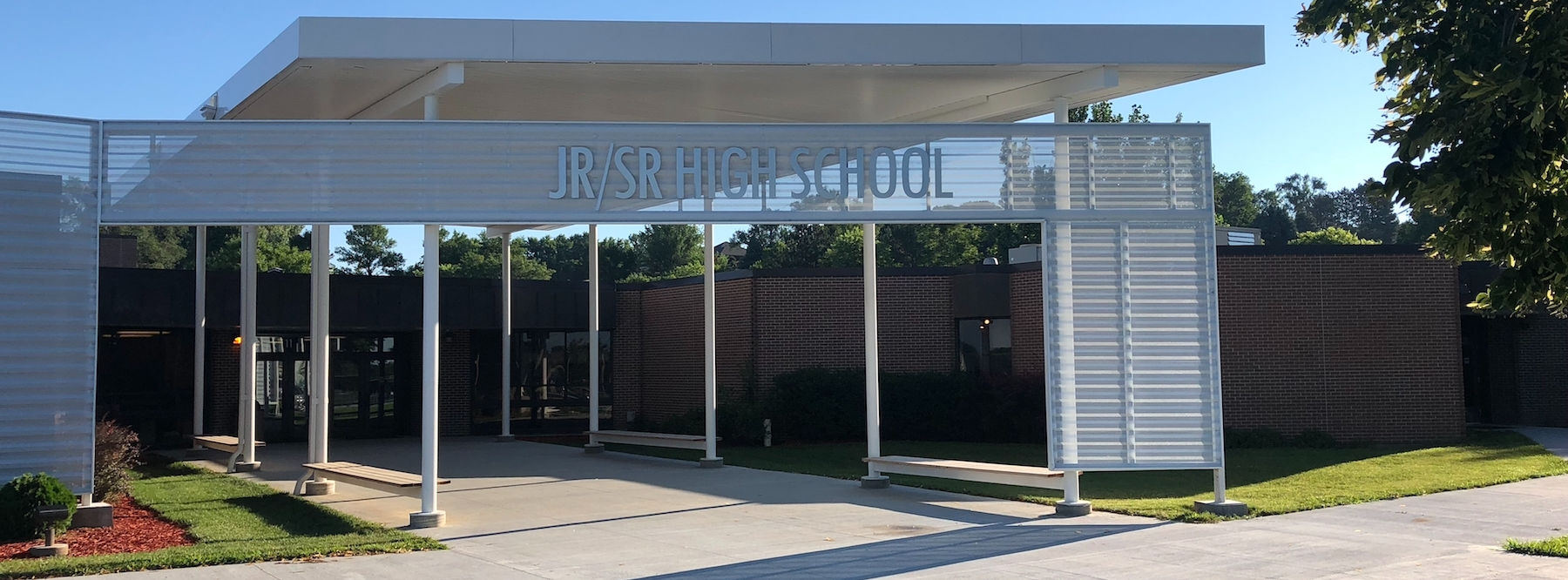The horizontal panoramic image depicts the entrance of a junior/senior high school building, characterized by its reddish-brown brick façade. The expansive concrete sidewalk in the foreground bifurcates, leading directly to the main doors at the center-left, while another path diverges to the right. The entrance is defined by a white awning or portico supported by pairs of white beams, creating a sheltered walkway. This awning features a prominent sign that reads "JR/SR High School" in white text against a rectangular backdrop.

Underneath the awning are four benches, each flanked by white supports that contribute to the structure's Venetian blind-like appearance. Surrounding the school’s entryway are neatly manicured lawns and neatly trimmed shrubbery, with areas of brown mulch providing a tidy contrast. Trees with lush green leaves frame the scene in the background, adding to the picturesque setting. The overall composition shows the school building in the right-hand portion of the image, highlighting the blend of natural and architectural elements. The bright white of the entrance structure stands out against the more subdued tones of the building and the greenery, creating a welcoming pathway to the school's main doors.